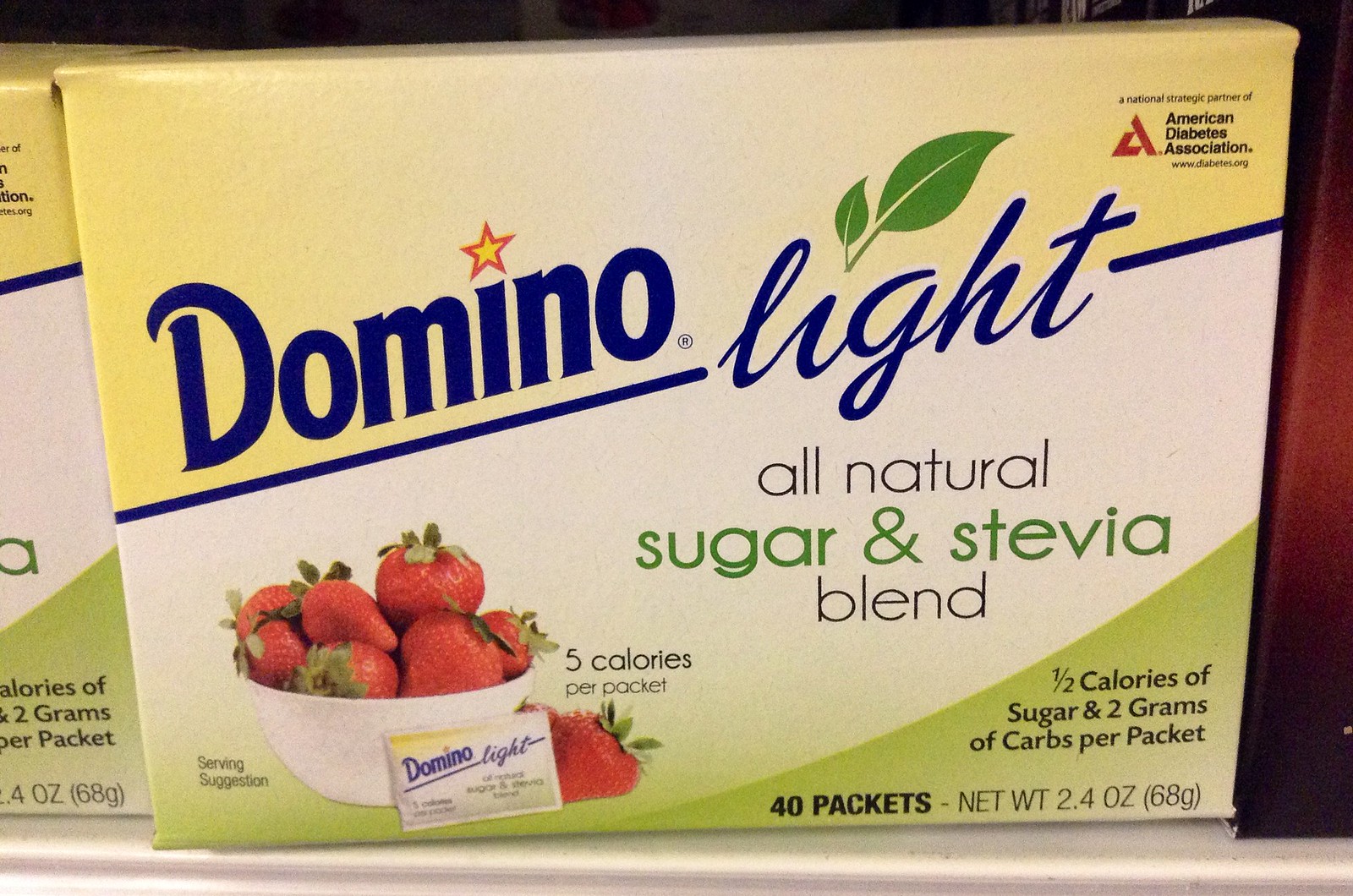This is a detailed close-up photograph of a yellow, white, and green box of Domino Light All-Natural Sugar and Stevia Blend, occupying almost the entire frame. Positioned on a store shelf, a silver border runs horizontally along the bottom of the image, with a distinct blue stripe separating the upper and lower sections of the box. To the left, partially visible, is the side edge of another box, featuring black lettering that reads “A-L-O-R-I-E-S, of, two grams, per pack, four ounces, and 68 grams.”

The main box prominently displays the brand name "Domino" in dark blue with a stylized star as the dot on the “i” and the word "Light" in cursive, accentuated with two green leaves. The top right corner features the American Diabetes Association logo, indicating its suitability for people managing diabetes. 

The bottom left section of the box depicts a detailed serving suggestion: a white bowl filled with strawberries, with additional strawberries placed outside the bowl. In the foreground, a small packet bearing the same "Domino Light" branding appears. 

The box highlights several product details in black lettering: "half calories of sugar and two grams of carbs per packet," "40 packets," "net weight 2.44 ounces," and "5 calories per packet." Additionally, the phrases "All Natural," "Sugar and Stevia Blend" are emphasized in white and blue lettering.